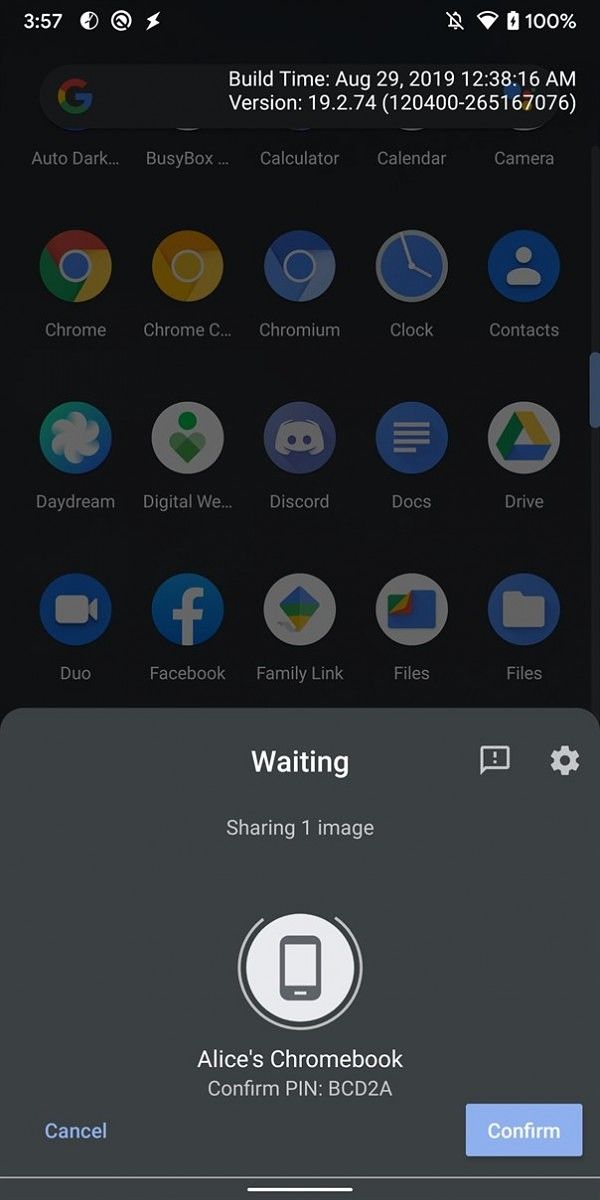The image depicts a predominantly black screen in a portrait orientation, resembling a mobile phone interface rather than a laptop. At the top, it displays typical clickable icons for launching various programs. The screen reads “Build date: August 29, 2019, 12:38:16 AM,” along with a version number. Most of the buttons are greyed out. Below, a smaller grey panel displays the message “Waiting” along with an information button and a settings button. Further down, the text indicates that one image is being shared. There is a round, white circle icon featuring a mobile phone in the center, which suggests that a photograph is being transferred either from a mobile phone to a Chromebook or vice versa. Beneath the icon, it reads “Alice's Chromebook,” accompanied by a prompt to confirm a PIN. The text shows “BCD2A,” and the “Confirm” button is highlighted, indicating that the process is currently underway.